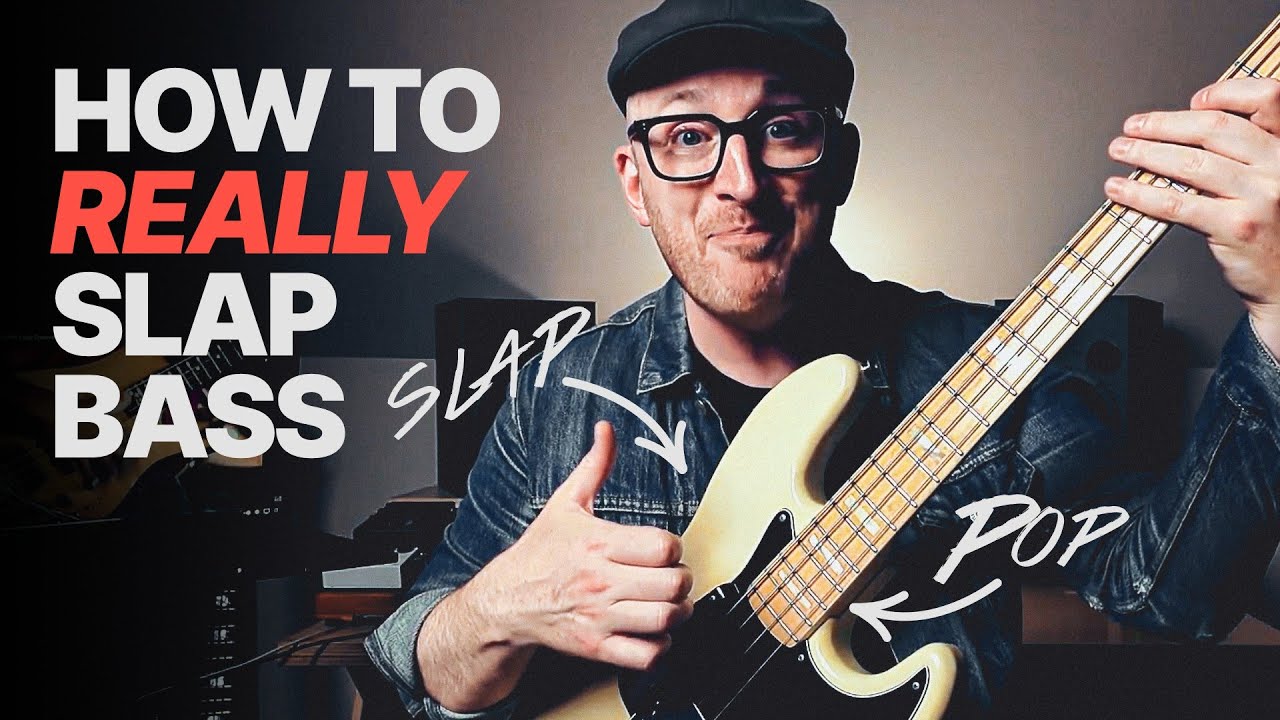The image depicts a musician situated in the center, holding a black and white bass guitar. He is a white male, wearing a blue jean jacket, black glasses, and a black beret. His eyes are wide open, and he appears to be semi-smiling. His left hand is positioned at the upper part of the strings, and his right hand is towards the lower portion. The backdrop features a white wall with a record player that is black, white, and brown, hinting at a modern setting.

Text on the screen appears in the upper left corner and reads "how to really slap bass," with "really" highlighted in orange while the rest of the text is in white. Additionally, the words "slap" and "pop" are written in white with arrows pointing towards the bass guitar, indicating a tutorial style aimed at teaching bass guitar techniques.